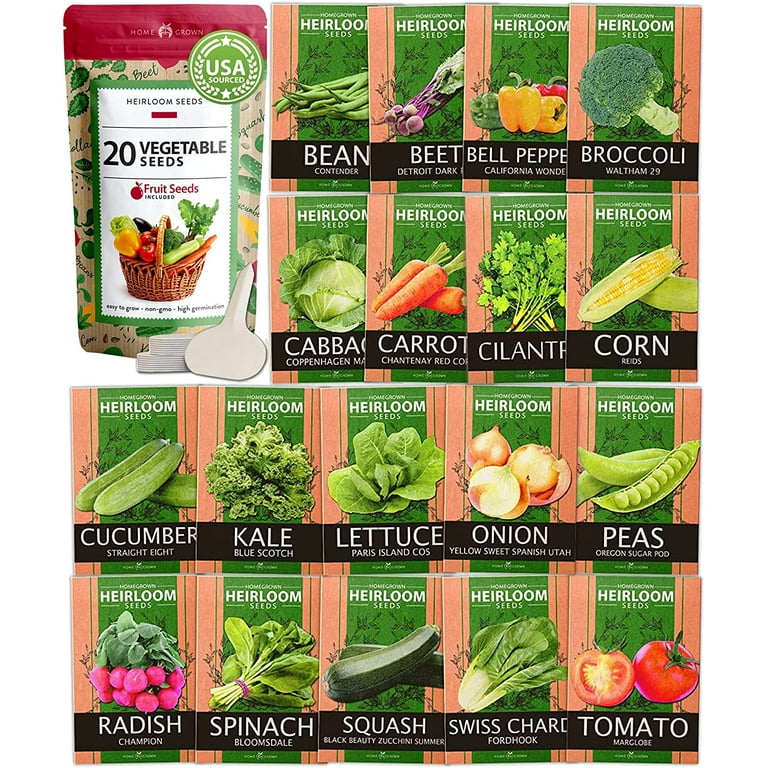This image is a detailed advertisement for a comprehensive packet of heirloom seeds. At the upper left-hand corner, the image features a red-bordered label that says "Homegrown," set against a brown and green leaf pattern. Central to the design, there is a stamp-like logo claiming "Heirloom Seeds" and denoting that the seeds are "USA Sourced." This section also shows a brown-handled wicker basket brimming with assorted vegetables such as yellow and green bell peppers, celery, kale, carrots, and broccoli.

The advertisement showcases 20 different types of vegetable seed packets, all nestled in an organized layout of four rows. Each packet is bordered in brown with a green interior, and a peach vertical stripe, featuring images of the respective vegetables. The top row includes packets for green beans, beets, bell peppers, and broccoli. The next row presents cabbage, carrots, cilantro, and corn. Following that are cucumber, kale, lettuce, and onions. The bottom row displays radishes, spinach, squash, Swiss chard, and tomatoes, with the latter showing a sliced tomato for clarity.

Additionally, there are small white signs provided to label the plants as they grow. These packets are all contained within a resealable main package, emphasizing convenience and organization for gardeners. This well-organized ensemble of seed packets aims to provide a rich variety of homegrown vegetables, reflecting detail in both its pictorial representation and labeling, affirming its heirloom quality.